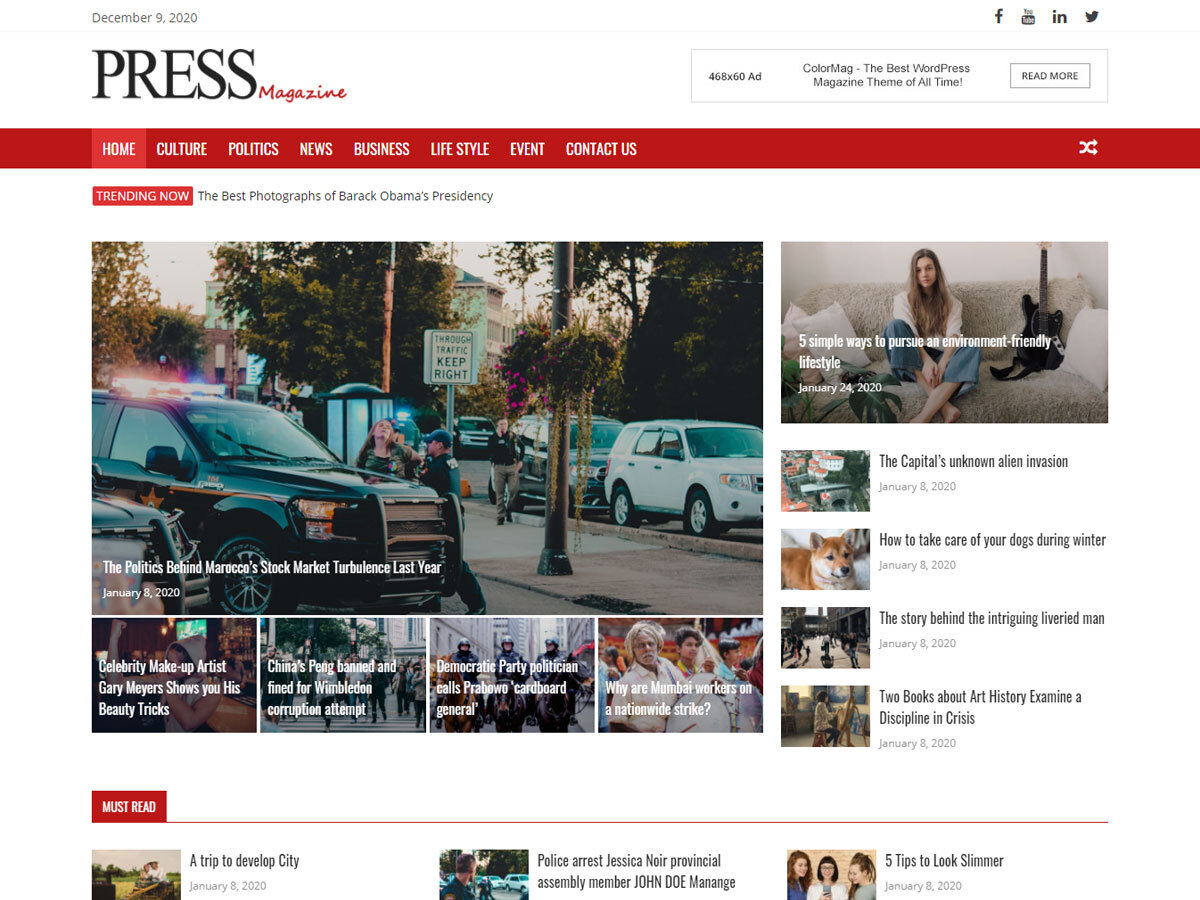Screenshot of an Online Magazine - December 9th, 2020

The screenshot is from an online magazine named "Press Magazine," featuring a red banner at the top with icons for Facebook, YouTube, Instagram, and Twitter (X) in the top left corner. The navigation menu includes options for Home, Culture, Politics, News, Business, Lifestyle, Event, and Contact Us. Below the menu, a red block marked "Trending Now" showcases "The Best Photographs of Barack Obama's Presidency." 

Beneath this block, various articles are highlighted with accompanying images. One image is a photograph taken outside depicting a policeman detaining an individual beside a black SUV cop car. The street is lined with park vehicles, including a white SUV and another black SUV. 

Another highlighted article features a woman sitting on a couch with a guitar, exuding a relaxed and creative ambiance. Additionally, there is an article with an image of a dog and a headline offering tips on "How to Take Care of Your Dogs During Winter."